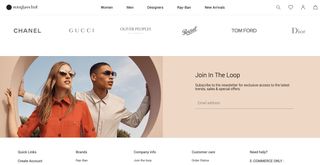This image features a highly blurred, low-resolution picture that required considerable zooming to view. The overall design showcases a luxurious theme. At the top, there is a decorative border listing several high-end brand names, including Chanel, Gucci, and Dior, set against a pristine white background. Above this border, there are some icons and a menu, while the top left corner displays an unidentified logo.

The central image shows a light-skinned woman with shoulder-length brown hair, posing against a light pink background. She is wearing a red, collared, long-sleeved shirt and sunglasses. Beside her stands a man who bears a remarkable resemblance to Barack Obama; he is dressed in a white, collared, long-sleeved shirt and also wears sunglasses.

To the right of this pair, the phrase "Join the loop" is prominently featured, followed by a text box presumably intended for users to input their email addresses. Unfortunately, some text within the image is too blurry to decipher. At the very bottom of the picture, another menu is visible, though its details are unclear due to the image quality.